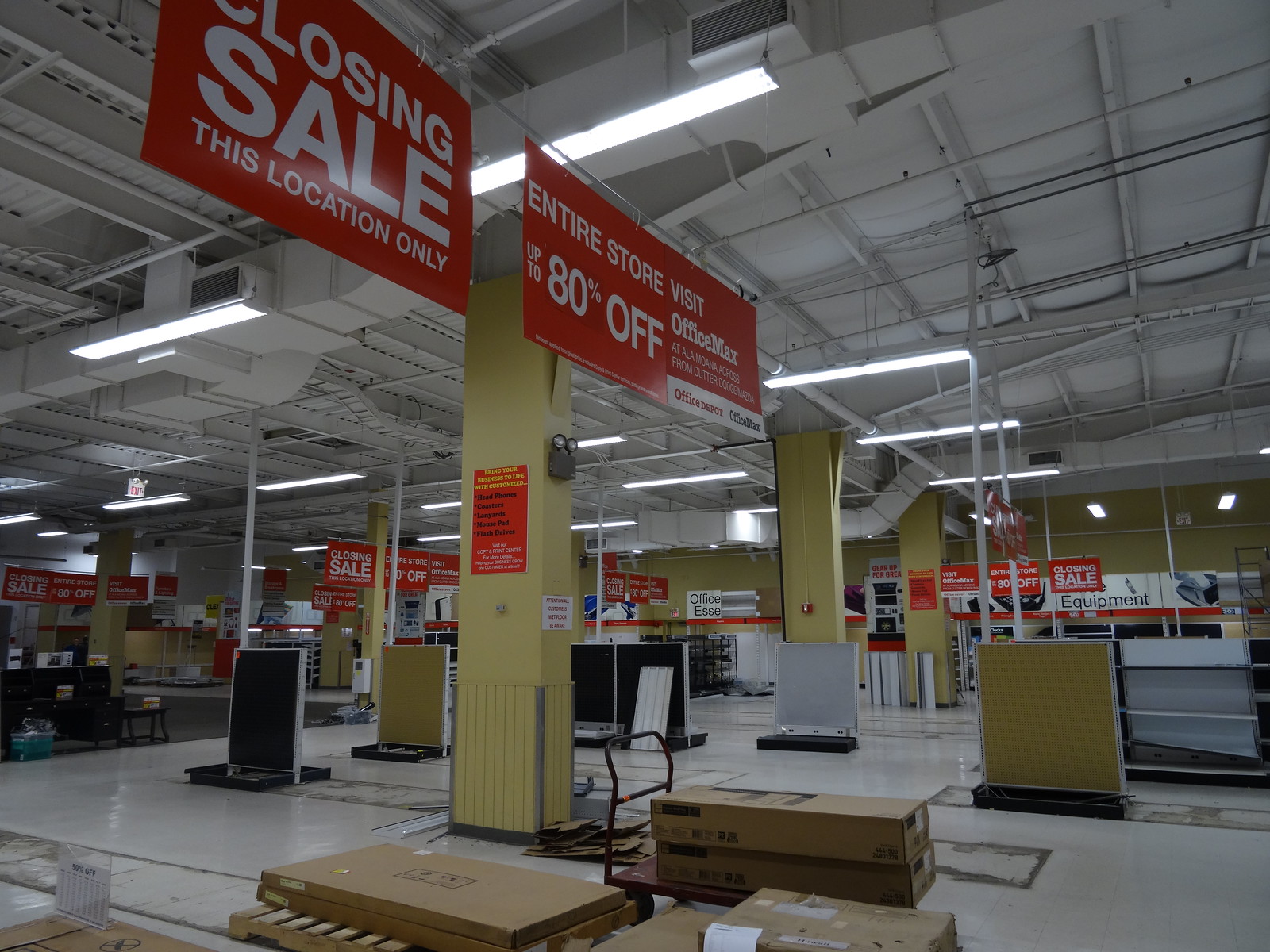This image captures the interior of a store that is in the process of closing down. The store is a vast, industrial-style space, characterized by its white-painted ceiling adorned with fluorescent lights. The floor, covered in highly polished white tiles, reveals scuffed and damaged areas where shelving units and displays once stood, now removed. Scattered throughout are numerous cardboard boxes, hinting at the packing and clear-out activities in progress. Two prominent red rectangular signs hang from the ceiling, announcing the closure: one sign declares "CLOSING SALE - THIS LOCATION ONLY," while the other advertises, "ENTIRE STORE UP TO 80% OFF - Visit OfficeMax." This scene poignantly captures the final days of a retail space.